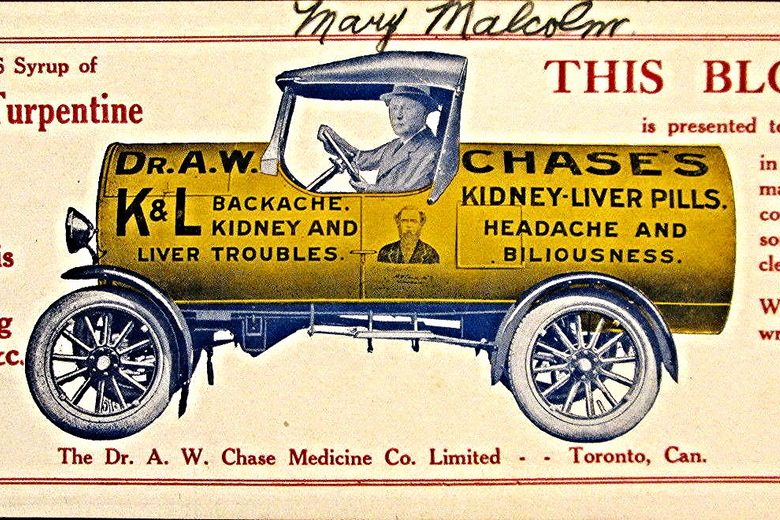This vintage advertisement features an off-white background, with "Mary Malcolm" elegantly written in cursive black script at the top. Dominating the center is an illustration of a man in a suit and top hat, confidently driving an old-fashioned car. Intriguingly, the body of the car is a cylindrical gold tank with black text, prominently displaying "Dr. A.W. Chase's Kidney, Liver, Pills, Headache, and Biliousness." On the left side of the tank, it reads "K&L Backache, Kidney, and Liver Troubles," while on the right side, it reiterates "Kidney, Liver, Pills, Headache, and Biliousness." The car features black and white wheels and has additional red text beneath it that states, "Dr. A.W. Chase Medicine and Company, Ltd., Toronto, Canada." The overall layout and style suggest it is a promotional piece from a bygone era, with meticulous details that capture the essence of vintage print advertising.